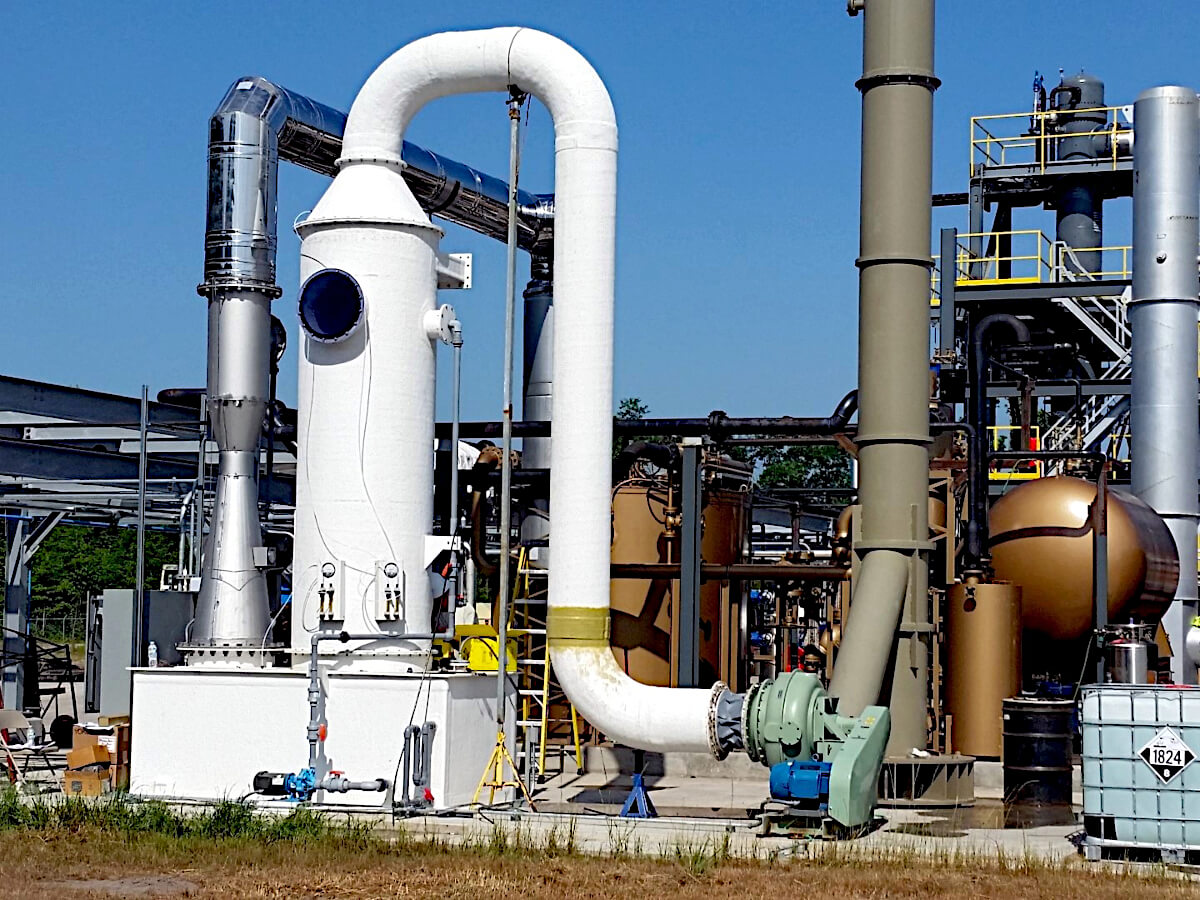This detailed photograph captures a bustling scene within a chemical refinery. Dominated by a complex array of pipes, this industrial area features piping in various hues - white, silver, beige, olive drab, and black - all set against a concrete surface with a strikingly blue sky in the background. Numerous chambers, gauges, dials, motors, and blowers are interspersed throughout the image, showcasing the intricate and essential instrumentation required for chemical processing. 

In the lower right, we see a round bronze-colored tank adjacent to a thick greenish-brown smokestack, reinforced at intervals with bolted rings, stretching upward and out of the frame. Nearby, a silver smokestack stands, accompanied by yet another dark gray one in the background, all connected by a network of external meters and instruments. A white pipe, curving up and looping back down into a large white tank with an open porthole, highlights the sophisticated engineering.

To the left of this setup, elevated catwalks and scaffolding lead up to platforms that interconnect these towering structures, with stairs extending three or four stories high. There's even a gentleman engaged in maintenance work around one of the white pipes.

A prominent feature in the scene is a small diamond-shaped black and white warning sign, labeled with the number "1824," hinting at the hazardous nature of the equipment. Large tanks, some upright and one lying down, add to the industrial landscape, while trees and the flawless sky in the background subtly contrast the heavy machinery. This photograph skillfully encapsulates the elaborate and dynamic environment of a chemical production facility.